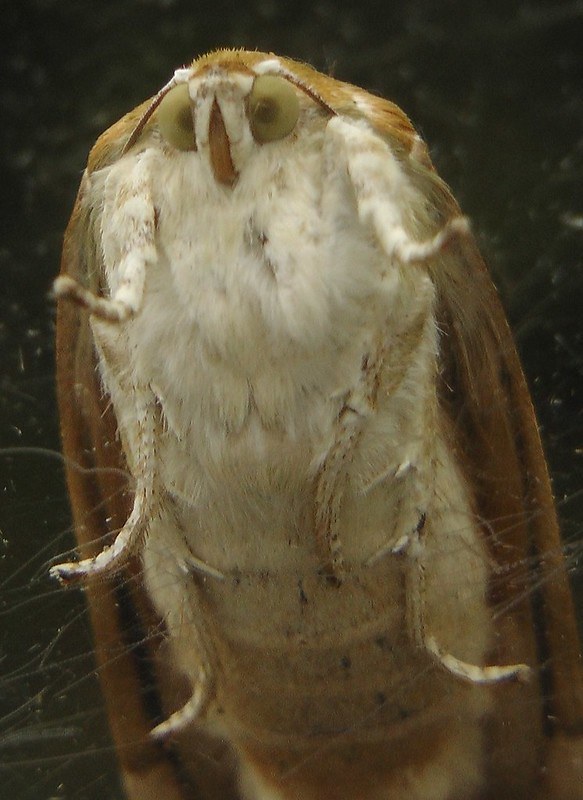This image showcases an extreme close-up of a large, furry moth, revealing intricate details that give it an almost otherworldly appearance. The moth is depicted with a chest and legs covered in what seems like soft, feather-like fur in shades of white, light brown, and spots of black. Its circular eyes, which have a light lime green hue, and a prominent, brown-colored nose-like structure are clearly visible. The moth's body, reminiscent of the shape and fur of a hamster, suggests it might be several inches to a foot long, with six legs and possibly wings that blend into its hairy form, making it difficult to discern if it can fly. The background of the image is mostly dark, with hints of green tones suggesting a forest setting. The photograph is characterized by scratches and dust, hinting that it might be a scanned print rather than a direct digital capture. The wings appear swept back, adding to the mysterious elegance of the moth against the blurred, dark background.